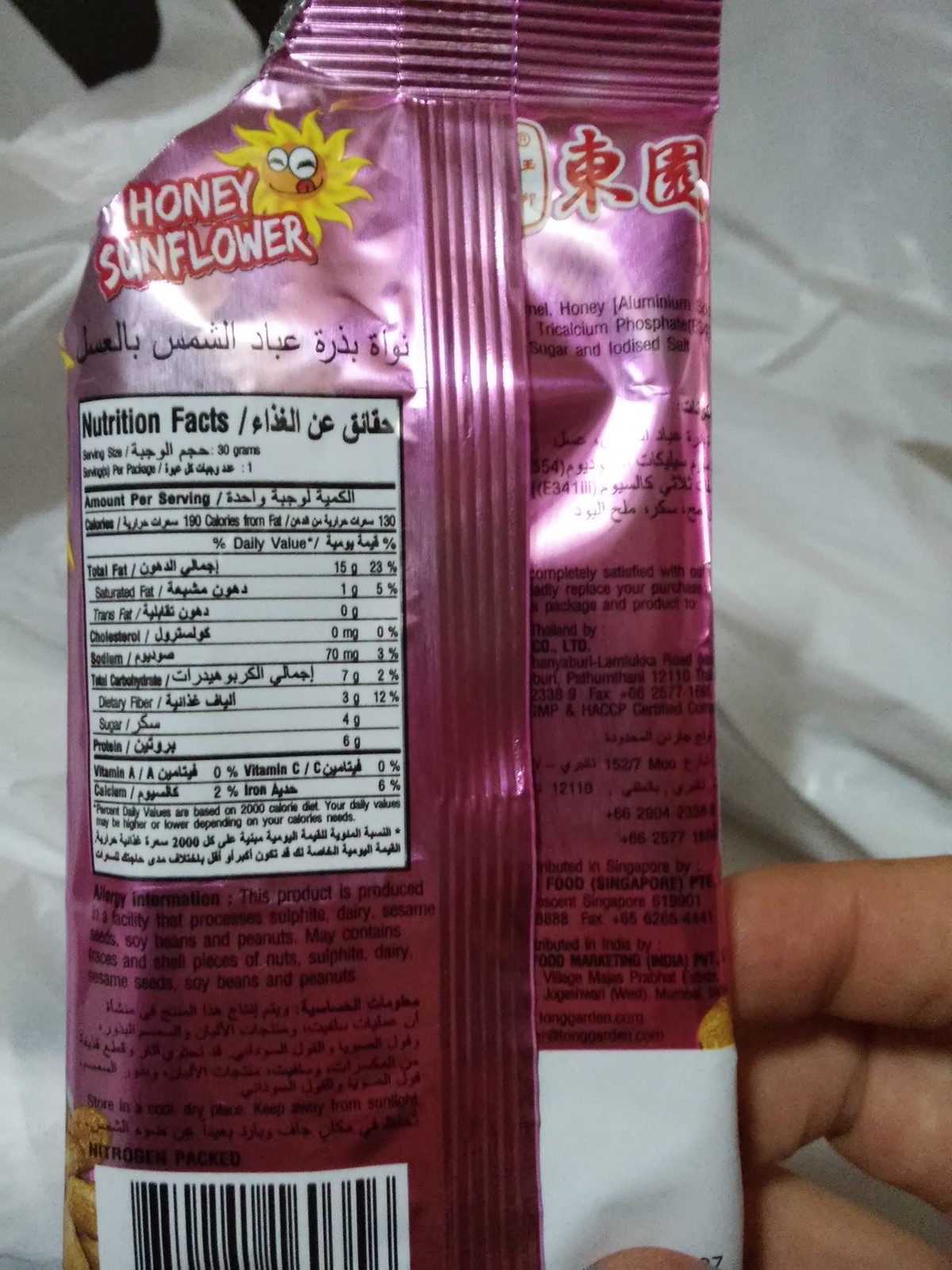The image captures the backside of a vibrant pink food package prominently featuring essential details about the product. The package displays nutrition facts, ingredients, and information about the company. The product is labeled "Honey Sunflower," accompanied by a whimsical illustration of a sunflower with a sun's face, complete with expressive eyes and a tongue playfully licking its lips. The packaging includes text in both English and what appears to be Japanese.

Highlighted ingredients in the list include honey, aluminum, sugar, and blue diced salt. Also visible are elements of the packaging origin details. A human hand is holding the package, providing a sense of scale and context. The backdrop of the image is plain white, possibly the bag that the package came from. Additionally, a barcode is clearly visible on the pink packaging, adding to the detailed informational display.